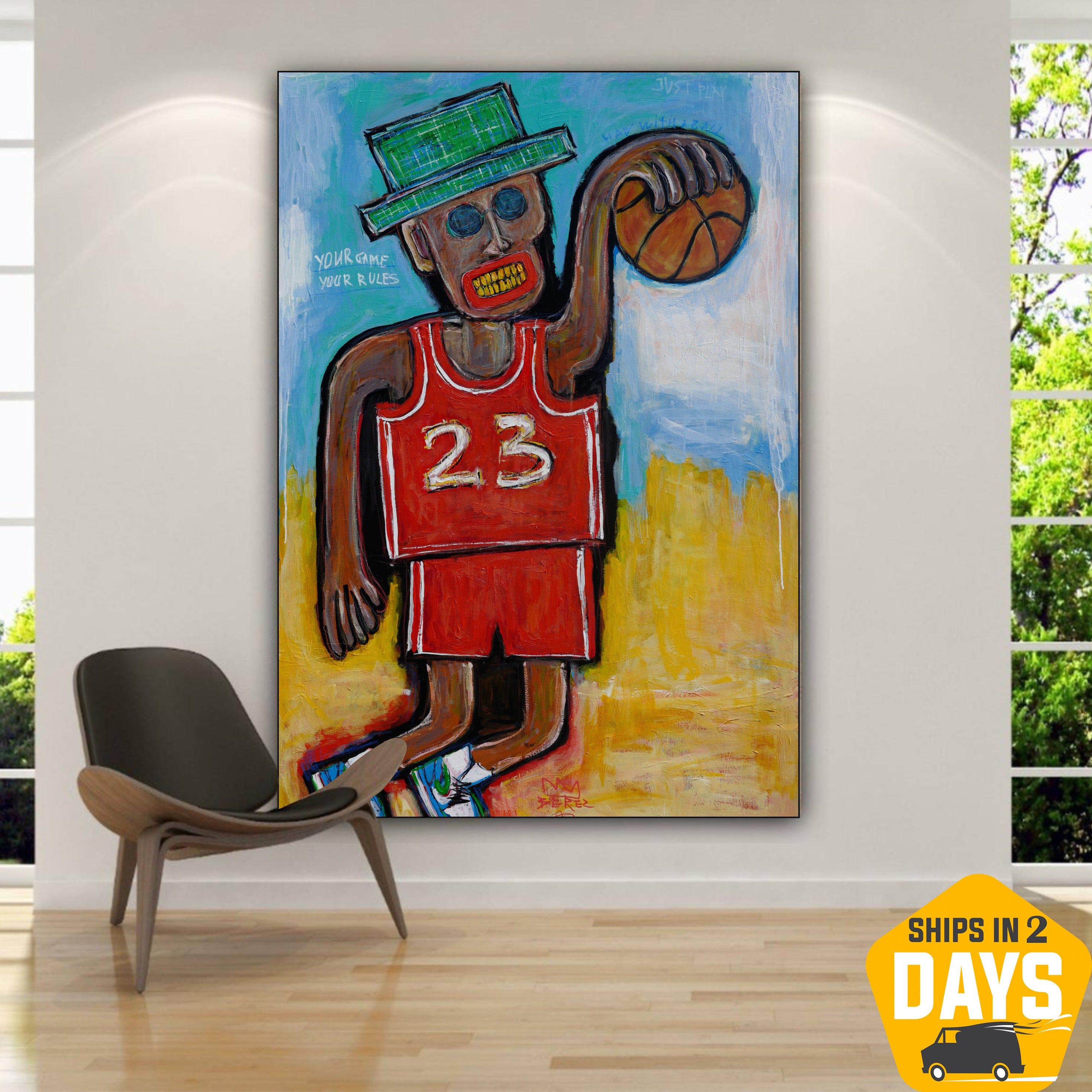This detailed description portrays a photograph of a contemporary room featuring a large, abstract, cartoonish painting of a character resembling Michael Jordan. The painting hangs on a white wall between floor-to-ceiling windows, revealing a room with wooden floors and a modern aesthetic, complete with a small chair in front of the artwork.

In vivid, exaggerated colors, the painting features an African-American basketball player in a red jersey and red pants with the number 23—Michael Jordan's iconic number. The player's appearance is highly stylized, almost eerie, with a skeletal face, deep eye sockets, and pronounced cheekbones. His big blue eyes poking out like buttons and yellow teeth contrast starkly with his red lips. He's depicted wearing a green hat adorned with red stripes, and he's palming a basketball in his left hand.

The background of the painting is a blend of bold blue and yellow paint strokes, infused with white streaks, creating an abstract and dynamic backdrop. Near the player's head, there's white text reading, "Your Game, Your Rules." At the bottom right corner of the painting is a small hexagonal logo with the phrase "Ships in Two Days" and an illustration of a cartoon delivery van.